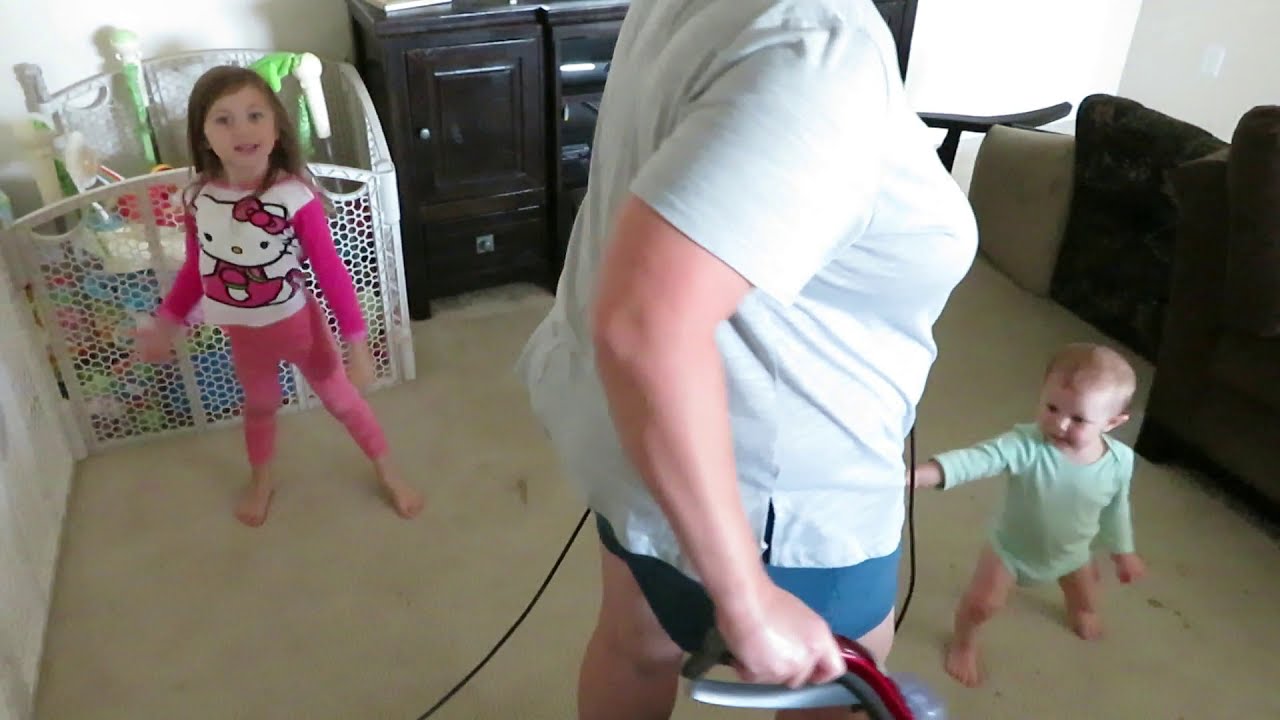In a cozy, well-lit living room with lighter-colored carpet and some dark furniture, a woman is captured in a high-angle shot while vacuuming the floor. She is wearing a white t-shirt and blue shorts, and although her face is not visible, she appears to be a bit heavy set. Behind her is a young girl, around 6 or 7 years old, dressed in a Hello Kitty pink sweatshirt and pink pants, with light brown hair. To the right of the woman, a toddler in a light green onesie, with sparse light brown hair, stands nearby, reaching out towards her as if offering help. The little girl is also looking up, perhaps at the person taking the picture. The room includes a black couch, a dark TV stand, and a playpen filled with toys, creating a warm family environment. The scene suggests a daytime setting, as natural light floods the room.